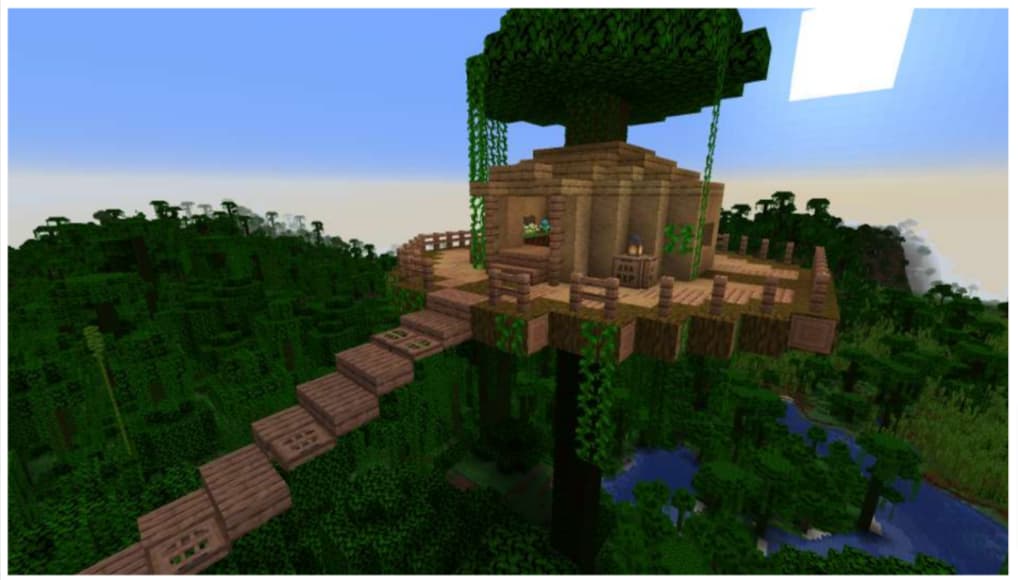This image, appearing as a screenshot from the game Minecraft, showcases a detailed pixelated treehouse nestled within a lush forest. The image features characteristic blocky, low-poly graphics indicative of Minecraft, with vibrant greens depicting stylized trees and leaves. At the scene's base, a body of blue water, likely a river, winds through the dense forest.

The main structure, an elevated treehouse, is a complex composition with brown steps sans rails leading to a multi-layered platform. This platform supports an open-air building with pillars, somewhat reminiscent of Aztec architecture. The treehouse appears to include various sections, possibly a main room with hints of yellow and green interiors, encircled by a deck.

A towering central tree, complete with cascading vines, extends from the platform, further contributing to the fortress-like feel. Outside the building, a lantern is perched on a small shelf, casting subtle light. The sky above is a flat blue with a large white square, potentially a stylized representation of a skylight or the sun. In the background, more pixelated green trees complete the immersive, blocky landscape. The image captures the essence of a serene yet meticulously constructed Minecraft world.